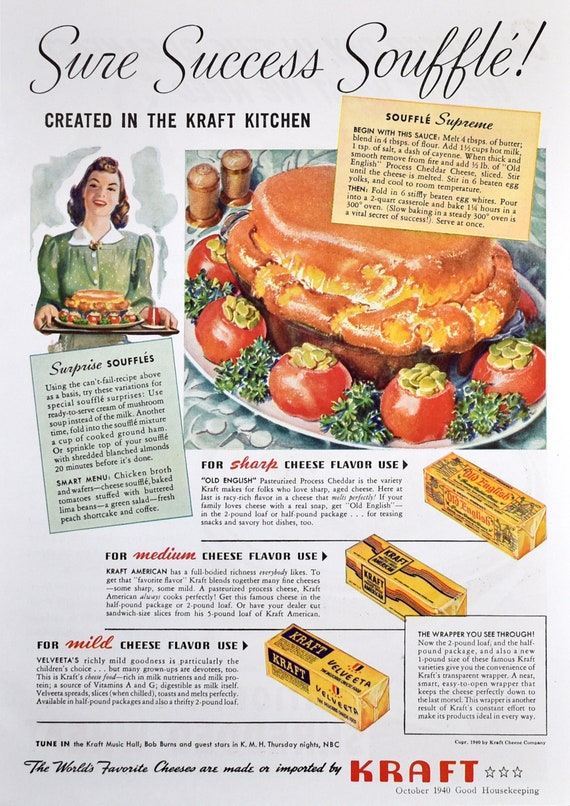This is a vintage 1940s magazine advertisement with a light gray background, primarily featuring a promotional poster for Kraft. The poster is titled "Sure Success Soufflé" in large black cursive text, with the subtitle "Created in the Kraft Kitchen" beneath it. On the left side, there's a watercolor-style illustration of a woman from the 50s era, wearing a green dress and holding a serving tray with a baked dish garnished with tomatoes. 

To the right of the woman, there's a close-up illustration of the same dish, showcasing a large golden brown pot roast surrounded by tomatoes and possibly lima beans. Below this, the advertisement highlights three types of Kraft cheese—sharp, medium, and mild—each represented by yellow blocks resembling butter sticks. 

The text on the poster is predominantly black, with certain keywords highlighted in red. At the bottom, the text reads, "The world's favorite cheeses are made or imported by Kraft," with "Kraft" prominently displayed in large red letters. The corner of the poster also features the publication details, indicating "Good Housekeeping, October 1940," further emphasizing its vintage style.